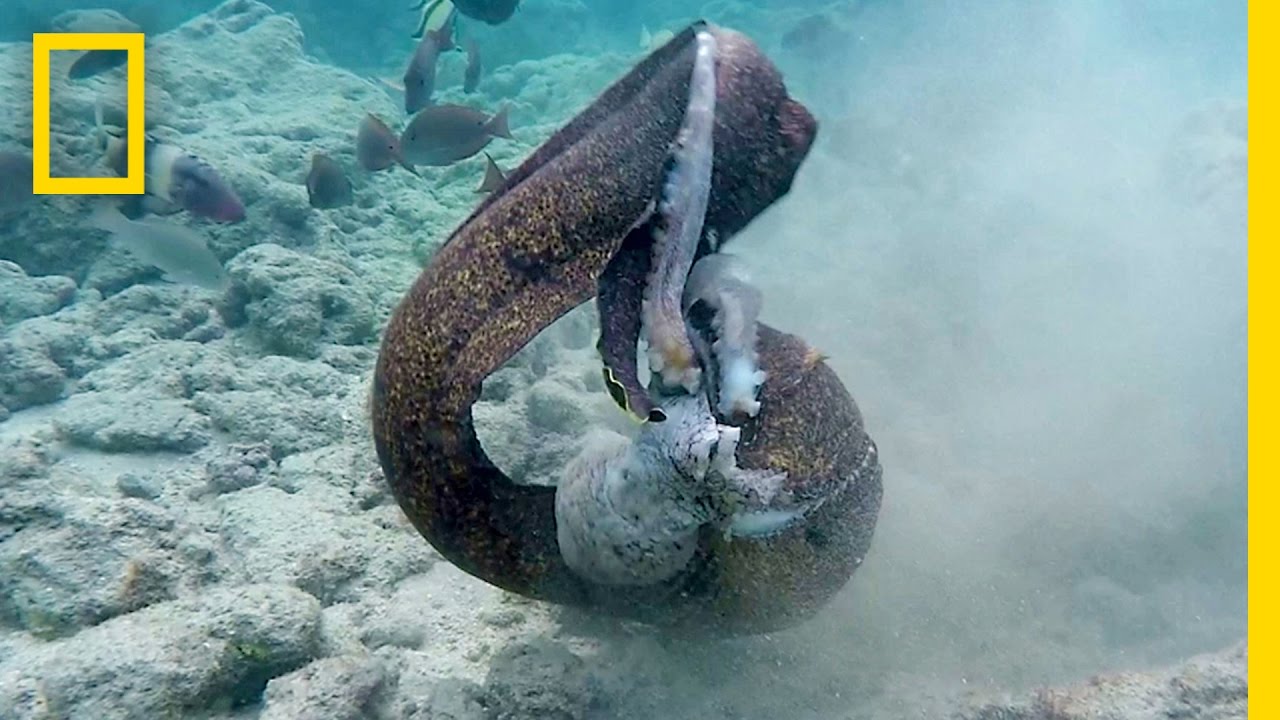This underwater color photograph, likely taken by National Geographic, showcases a mesmerizing aquatic scene. Dominating the foreground is the bluish-gray, tan-speckled limb of an octopus, featuring three distinct bends that shape it into a snake-like form. The arm, possibly severed and still reflexively mobile, intricately wraps around a light blue, unevenly textured object resembling a ball of dough. Beneath this interaction lies a sea floor comprised of light blue, pitted rocks. In the murky background, a dispersed school of dark blue-gray fish swim, seemingly indifferent to the scene. On the right side of the image, a cloudy white mist blurs the view, contributing to the mysterious underwater ambiance. The iconic yellow rectangle of the National Geographic logo is distinctly visible in the upper left-hand corner, framing this captivating marine tableau.